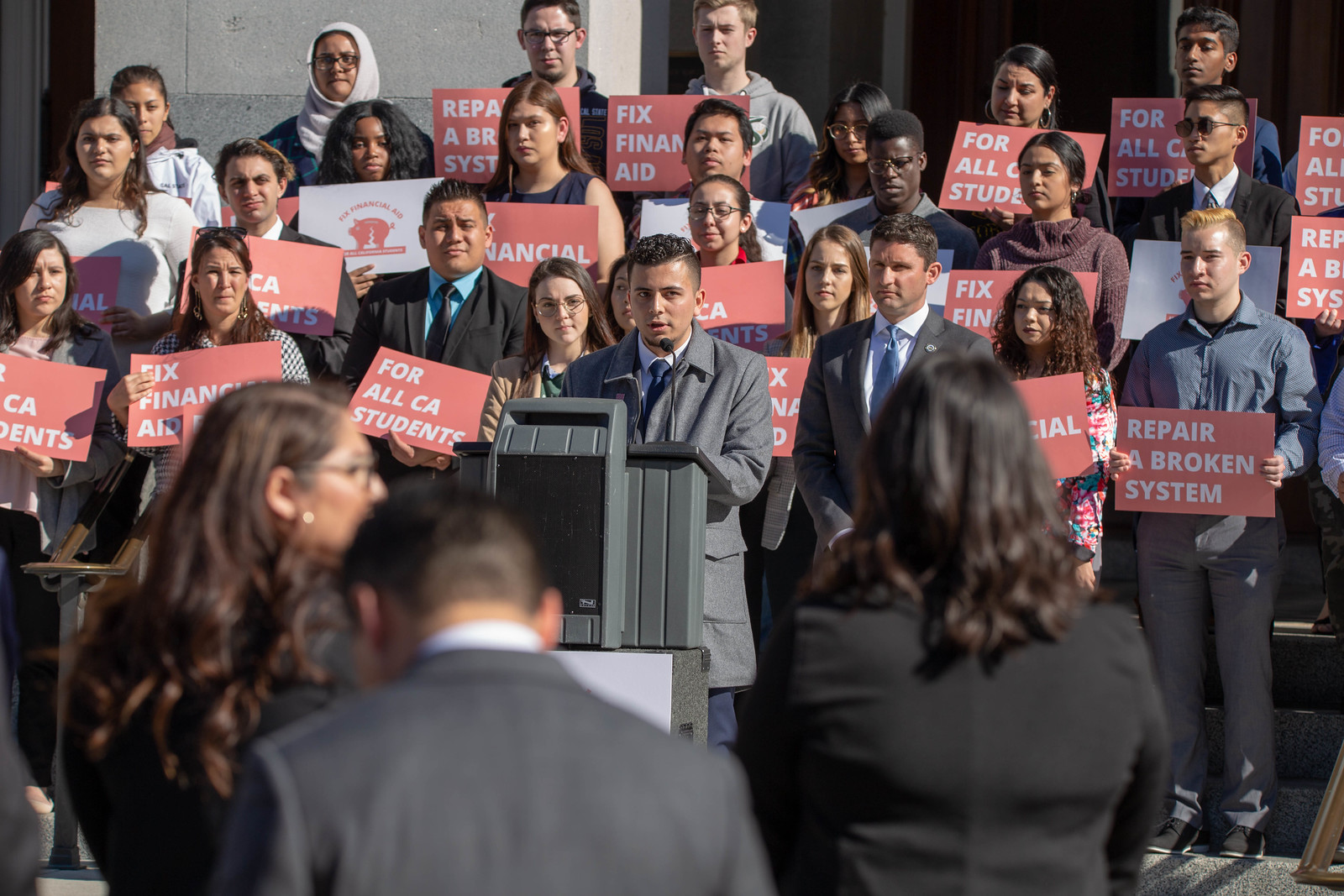The photo captures a professional protest scene outdoors in the middle of the day. Central to the image, a young man in a gray dress jacket, blue tie, and button-down shirt stands at a futuristic-looking podium, addressing the crowd with a microphone. Surrounding him are people of diverse backgrounds, all dressed in formal attire, including men in suits and ties. They hold peach-colored signs with white writing that convey messages such as "Repair a broken system for all California students," "Fix financial aid," and "Fix the system." The arrangement of the crowd suggests an elevation effect, as if they are positioned on steps behind him, giving depth to the image and highlighting the collective call for educational reform. The color palette includes shades of black, dark gray, light gray, orange, red, brown, and white, adding to the visual diversity of the scene.